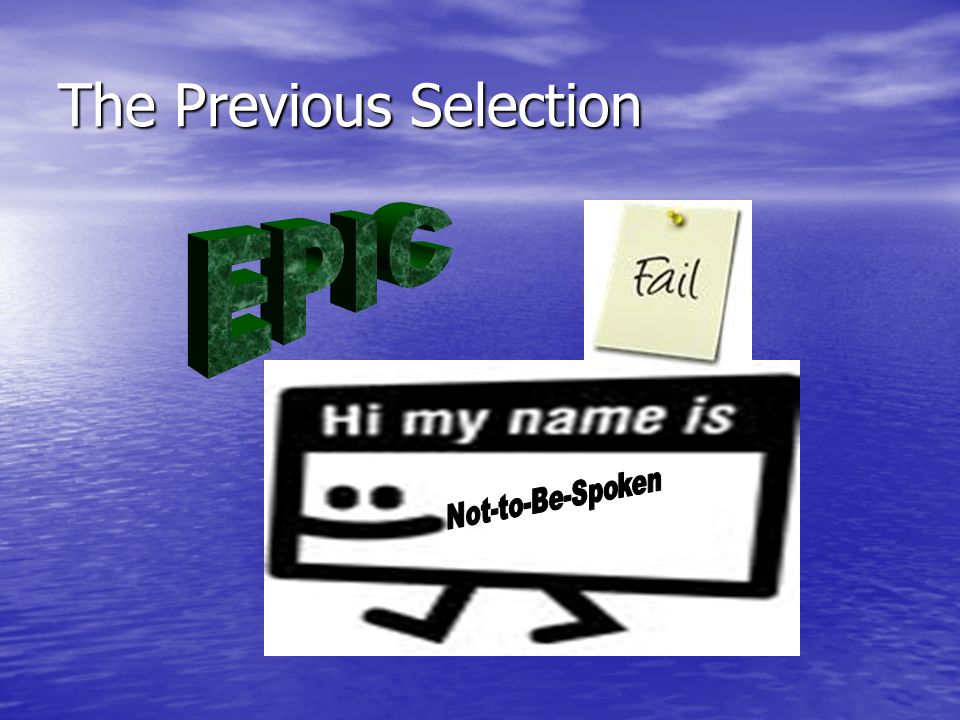The image is a Photoshop collage that merges photography, illustration, and typography with a distinctly 90s aesthetic. The background features a bright blue ocean occupying the lower three-quarters of the image, topped by a horizon of white mist that extends from left to right, accented with a light source at the left center. Above this, a blue sky dotted with thin white clouds forms the upper section. In the sky, white text reads "the previous selection." Below this, layered over the ocean on the left, the word "epic" appears in a green marbleized 3D font with a black drop shadow. To the right, a note that looks like it’s pinned up says "fail" in black handwriting. Beneath these elements is a vintage-styled name tag graphic that reads "Hi, my name is" followed by a smiley face and the text "not to be spoken." The tag features two stick-figure-like feet beneath it, suggesting motion. The overall composition combines photographic realism with retro typography and illustrative elements, creating a visually eclectic and nostalgic scene.